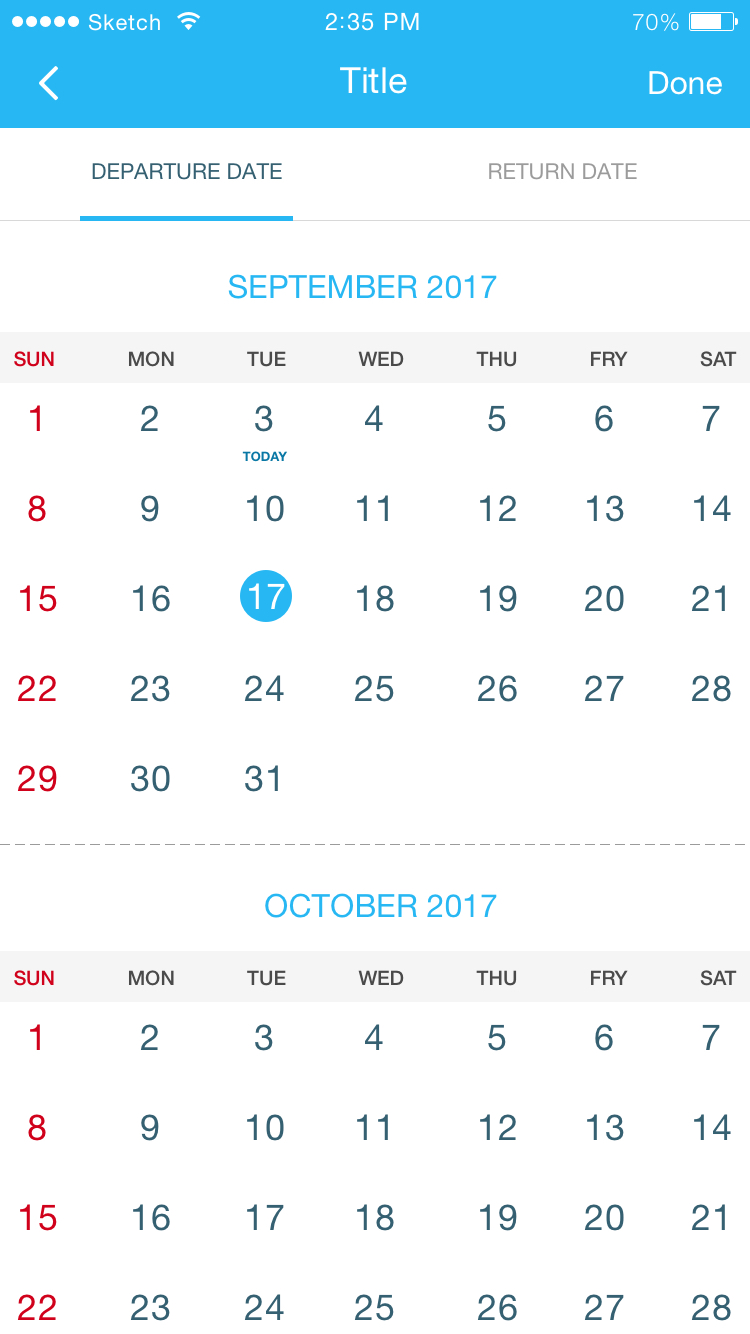This image is a screenshot from a phone, detailing various on-screen elements. At the top, a blue status bar displays the current time as 2:35 p.m. with white text. On the right side of this bar, the battery icon shows 70% charge remaining. On the left side, "Sketch" is displayed as the name of the mobile network, alongside icons indicating signal strength and an active Wi-Fi connection.

The main portion of the screen features a travel website's calendar interface. Two months are visible: September 2017 and October 2017. The 17th of September is specifically highlighted, suggesting it may be the selected departure date. The interface consists of two tabs; the "Departure Date" tab is currently active and highlighted, while the "Return Date" tab remains inactive and greyed out below.

The screenshot thus captures detailed phone status information and a travel calendar interface, providing options to pick departure and return dates, with the 17th of September 2017 highlighted as a significant travel date.